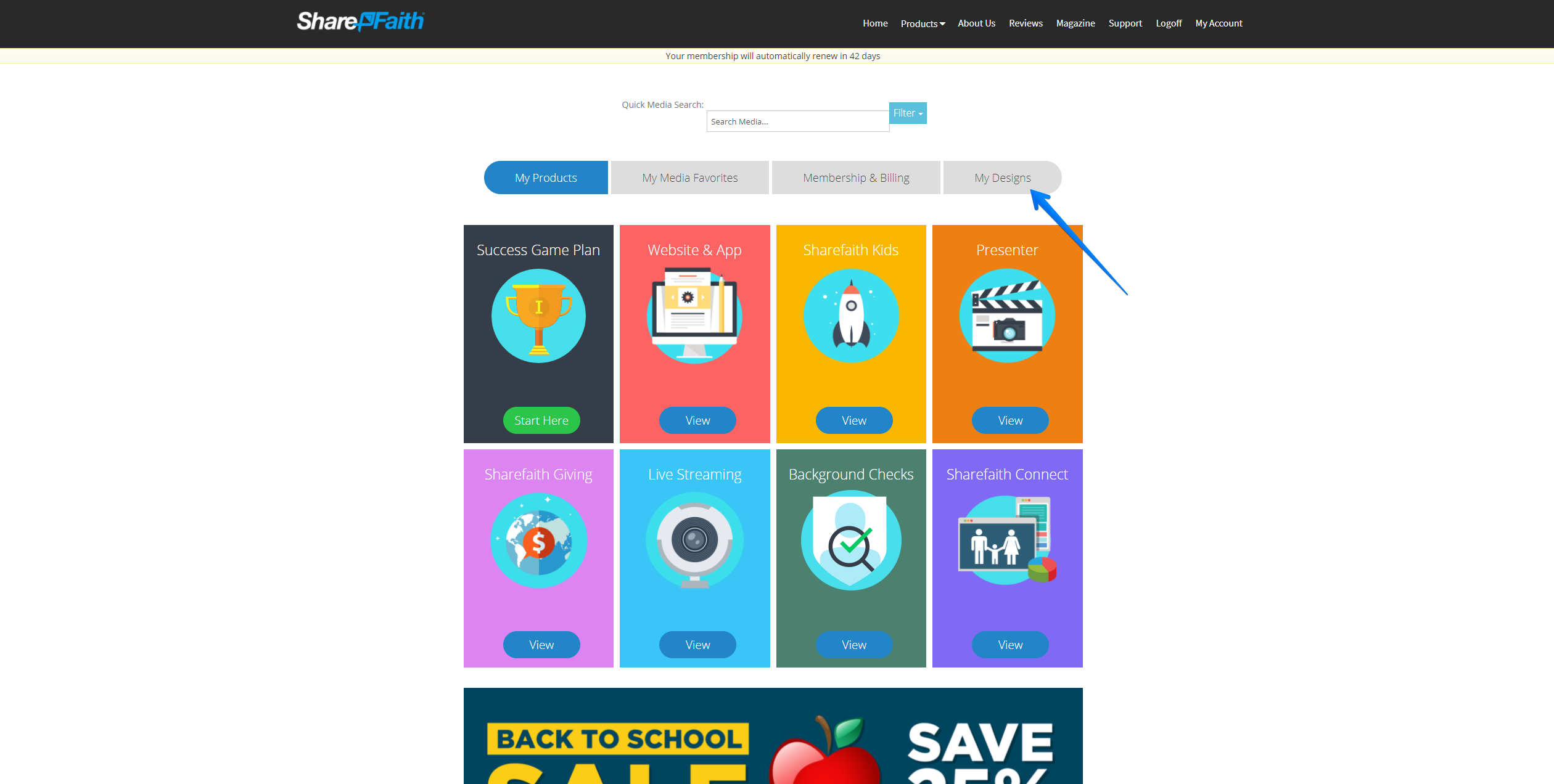This image is a screenshot from a website or app interface. At the top, there is a prominent black banner featuring the company's logo, "ShareFaith." The logo consists of the word "Share" in white and "Faith" in blue, separated by a stylized blue fish symbol. Towards the right side of this black banner are various navigation options: Home, Products (with a drop-down arrow), About Us, Reviews, Magazine, Support, Log Off, and My Account.

Beneath the black banner is a thinner gray banner containing an alert message, "Your membership will automatically renew in 42 days."

Following this, there's a search area labeled "Quick Media Search," including a search bar that says "Search Media" and a filter drop-down option on the right.

Directly below the search area is a navigation row with tabs named My Products, My Media Favorites, Membership and Billing, and My Designs. A blue arrow points to My Designs, emphasizing it, while the My Products tab is highlighted in blue, indicating it is the currently selected tab.

Further down are two rows of categorized links. The top row includes Success, Game Plan, Website and App, ShareFaith Kids, and Presenter. The bottom row lists ShareFaith Giving, Live Streaming, Background Checks, and ShareFaith Connect.

At the very bottom, partially cut off, is a promotional banner for a Back to School Sale, featuring an image of an apple, the word "Save," and partially visible percentage discounts.